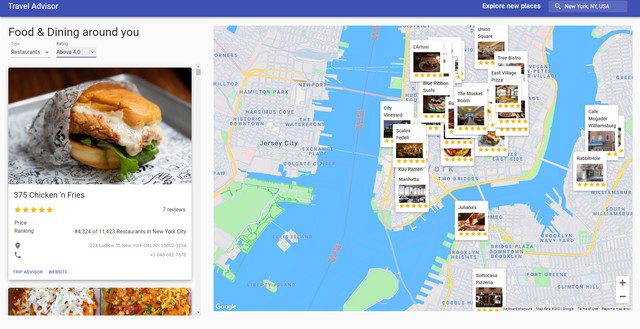The image features a webpage layout with a distinct blue bar running across the top. The bar includes the text "Travel Advisor" in white on the left side, while the right side prompts "Explore new places?" followed by a search bar currently displaying "New York, NY, USA." Below this bar, the page is divided into two main sections.

The left one-fourth of the layout presents a rectangular section titled "Food and Dining Around You." Within this section, there's a picture of a sandwich, possibly a chicken sandwich with sauce and lettuce, nestled in a bun. Accompanying this image is text indicating the meal's price: "$3.75 Chicken and Fries." Below this, two smaller rectangles feature images of pizzas, allowing for additional culinary options. A scroll bar is available for navigating through more images and information.

The remaining three-fourths of the page is occupied by a detailed map, illustrating three islands that make up parts of New York and extending into some areas of New Jersey. Various waterways separate these landmasses. The New Jersey section is devoid of icons, whereas the central and right-side islands in New York display several markers that point out different restaurants.